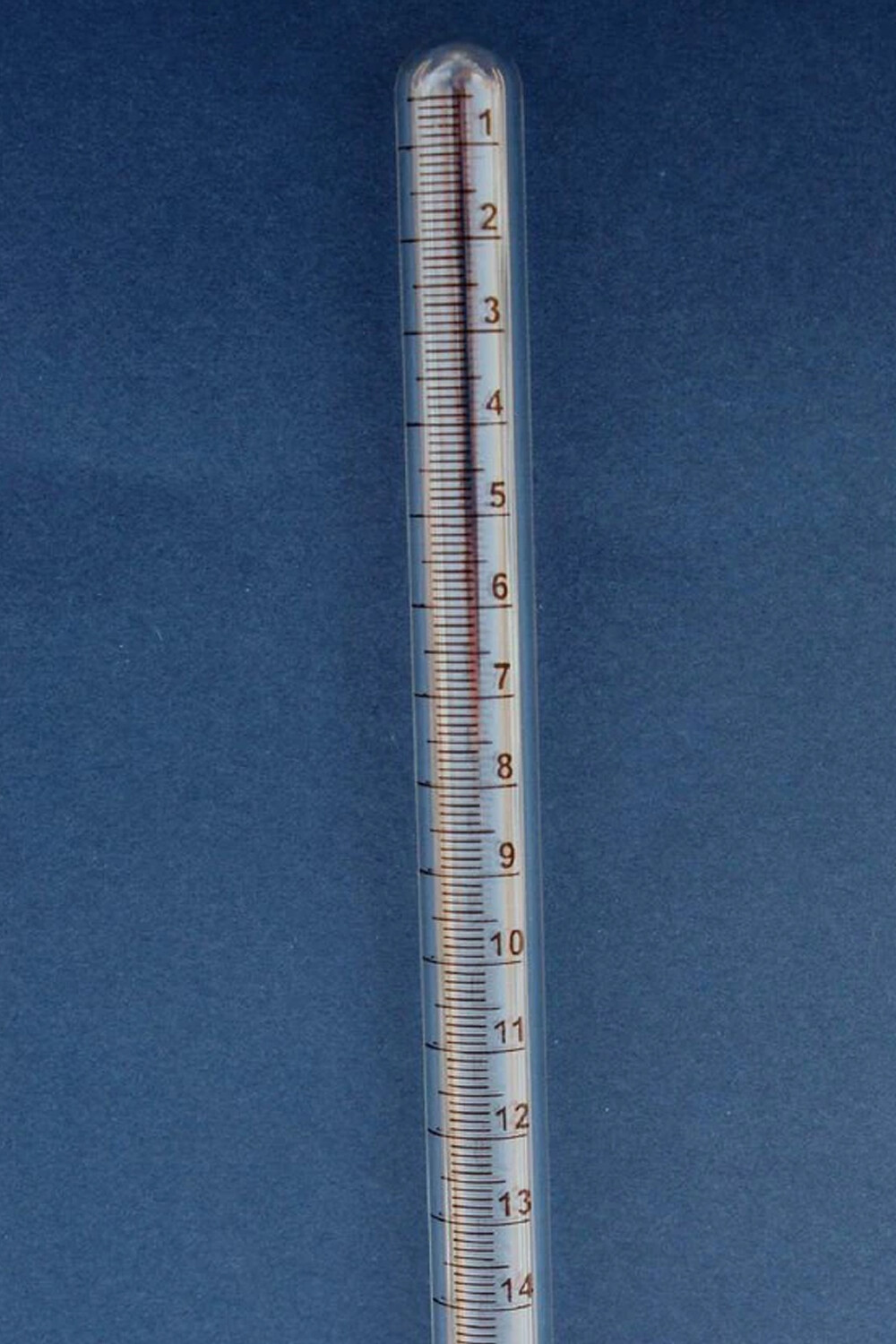In this image, there is a prominent thermometer centered at the bottom, set against a blue background that is marred by a significant amount of dust and artifacts. The thermometer is clearly marked with a scale that ranges from 1 at the top to 14 at the bottom, with numerous dash marks delineating each unit. This scale is meticulously detailed, showing every division from 1 to 14. The liquid inside the thermometer rises up to the 7 mark, indicating its measurement. The image quality is notably low, which adds to the overall dusty and artifact-filled appearance. Additionally, the blue background features subtle variations in shade, with lighter hues appearing toward the bottom left and bottom right, and darker tones occupying the top left and top right corners.